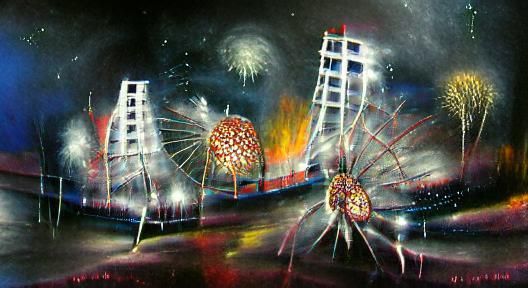The image presented is an abstract painting with a distorted, surreal quality. Dominating the scene are two white, skyscraper-like structures with red accents at their tops, positioned upright near the center. The background is a chaotic mix of deep blacks, blues, and reds, interspersed with bright patches of yellow and white, evocative of fireworks or a galaxy-like night sky. The lower portion of the image reveals a black pavement that reflects these vibrant colors, giving the impression of wetness. Additionally, warped elements suggest a central point of distortion, as if the image has been struck, resembling shattered glass. Amidst this tumultuous setting, there are vague figures—possibly spidery creatures or crustaceans with mottled red and yellow bodies and elongated appendages—engaged in a confrontation. The entire scene evokes a nightmarish, almost otherworldly landscape, blending elements of reality with an unsettling, abstract interpretation.